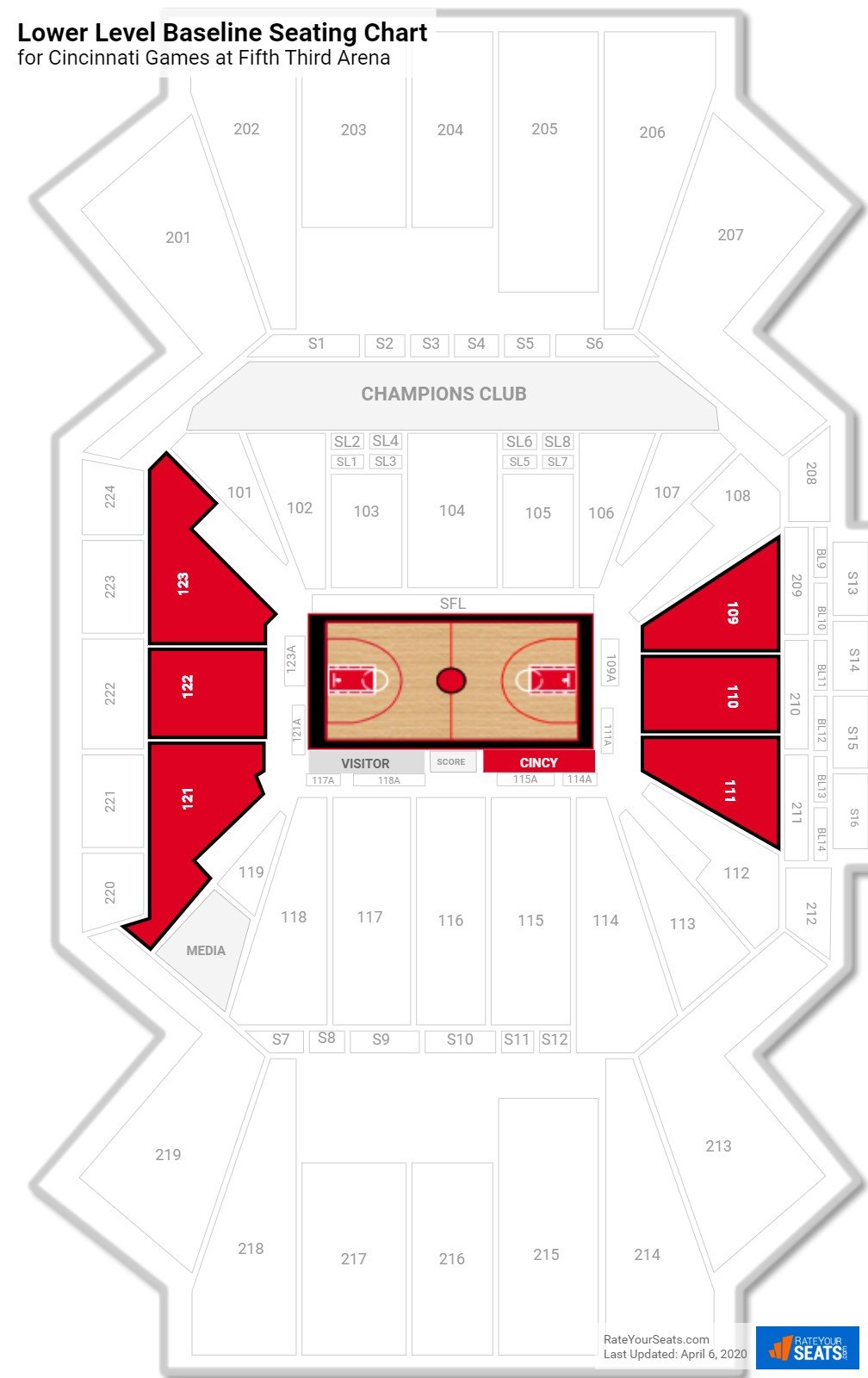This image depicts a detailed seating chart for the lower level at the 5th Third Arena in Cincinnati, specifically for an upcoming basketball game. Prominent red sections highlight premium seating areas: there are designated court-side boxes with three on each side of the court, although one side features two significantly larger boxes. The Champions Club area is also marked but does not have dedicated seating, suggesting it is a standing-room section for exclusive viewing. This comprehensive lower-level seating layout emphasizes the prime locations and facilities available for spectators during the Cincinnati basketball game.